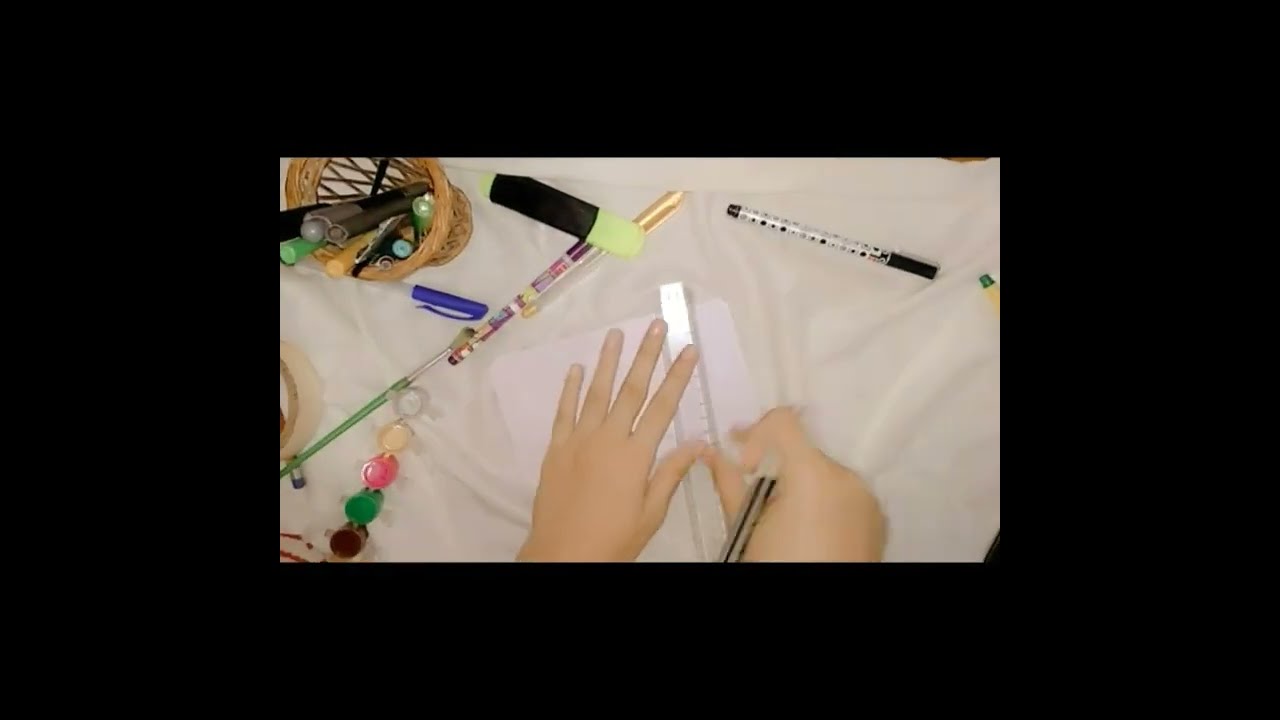The image depicts a close-up of a person's hands engaged in an arts and crafts project on a white surface. The person is using a clear plastic ruler and a pen to stencil or draw precise lines on a thin material, possibly clear plastic or paper. Surrounding the main activity area, there are various art supplies: to the left, there is a set of small paint containers in shades of brown, green, pink, beige, and white, accompanied by a green-handled paintbrush. A blue marker with a blue cap and a black pen with polka dots are also visible. In the upper left corner, a small wicker basket filled with assorted pens and markers is seen. The scene is framed by a thick black border, suggesting it might be a screenshot from a video.